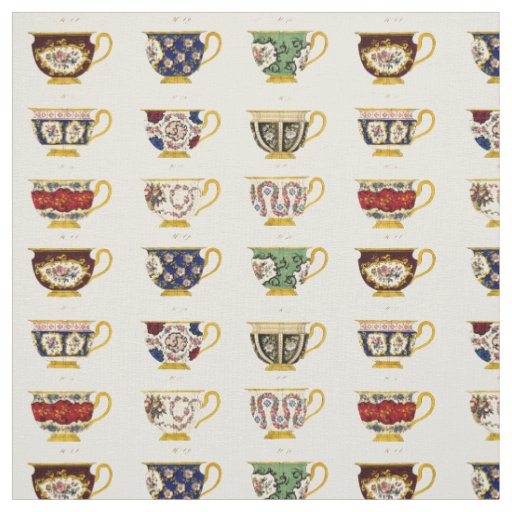The image depicts a detailed pattern of teacups arranged in several rows on a completely white background. Each teacup features intricate floral designs in a variety of colors, including brown, blue, green, black, white, red, pink, and orange. All the teacups are illustrated with marker and watercolor, showcasing a mix of colors such as yellow, gray, and blue with pink flowers. Additionally, they all have uniform gold handles, rims, and a gold base. Among the designs, some teacups stand out with dragon illustrations, providing a unique touch. The arrangement is such that the pattern repeats every few rows, with each teacup having its specific place in the sequence: a blend of brown, blue, green, and multicolored teacups distributed evenly across the image.